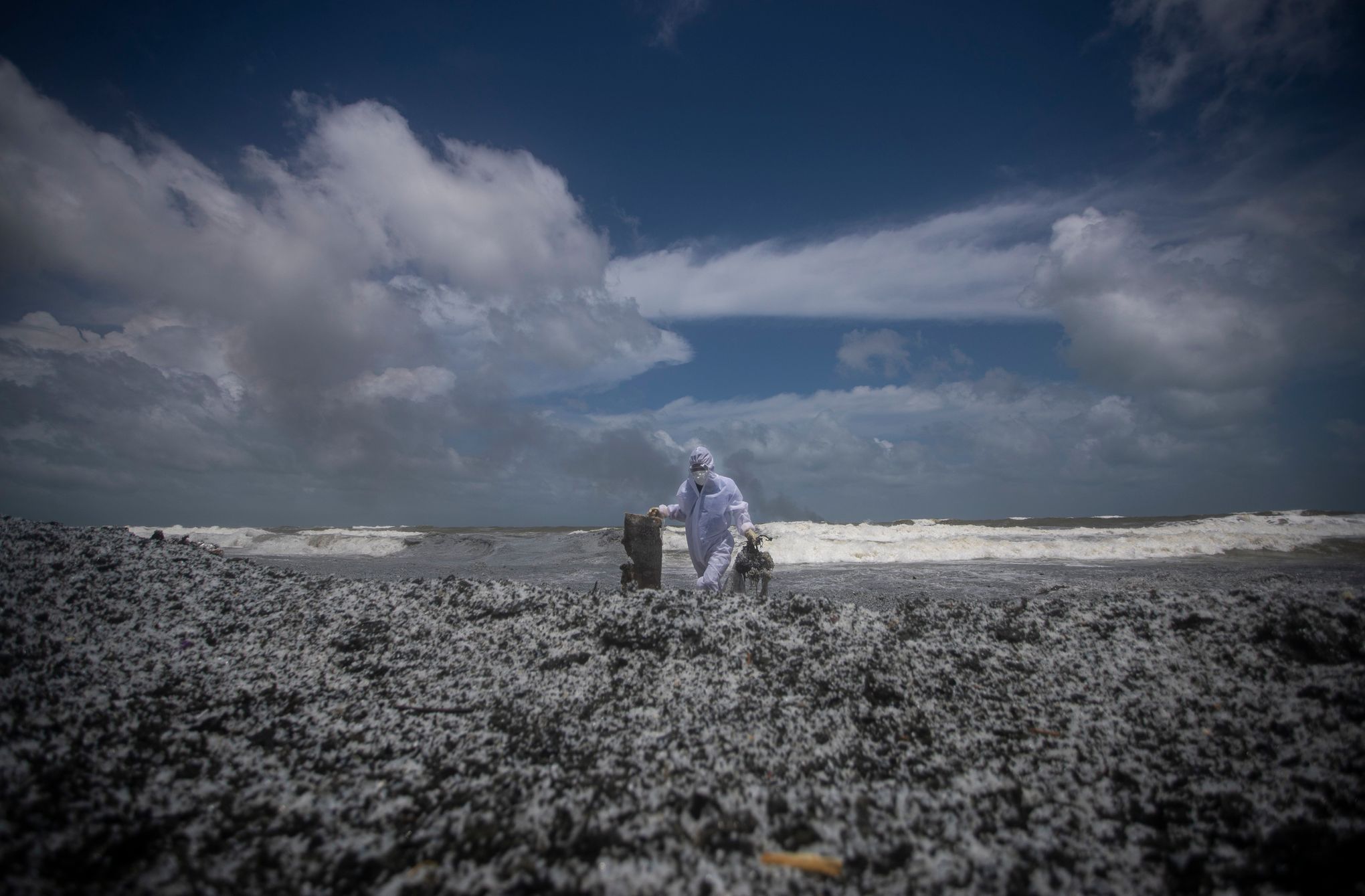In the image, a solitary figure stands at the convergence of a rugged shoreline and a turbulent ocean. The expansive blue sky, filled with wispy and deep gray clouds, dominates more than half of the picture, creating a striking contrast with the scene below. Choppy waters with thick, white-capped waves crash onto the shore, blending seamlessly with the rough, granite-like terrain that occupies the lower portion of the photo. This stony terrain varies in color from dark gray to black, overlaid in parts with a white, snow-like coating, possibly indicating frothy surf or remnants of a recent tide.

At the very center of the image is a person whose gender is indeterminate, dressed in a loose-fitting, all-white outfit that resembles a sanitation jumpsuit. They wear a white hood, face mask, and a white hair net, giving them an almost spectral appearance against the stark background. The figure appears to be holding two objects, one in each hand, potentially debris or pieces of trash, suggesting they might be engaged in cleaning efforts, possibly from a recent oil spill. The figure’s presence, combined with the desolate and somewhat blurry quality of the photograph, conveys a profound sense of isolation and dedication amidst the natural, yet harsh, coastal environment.